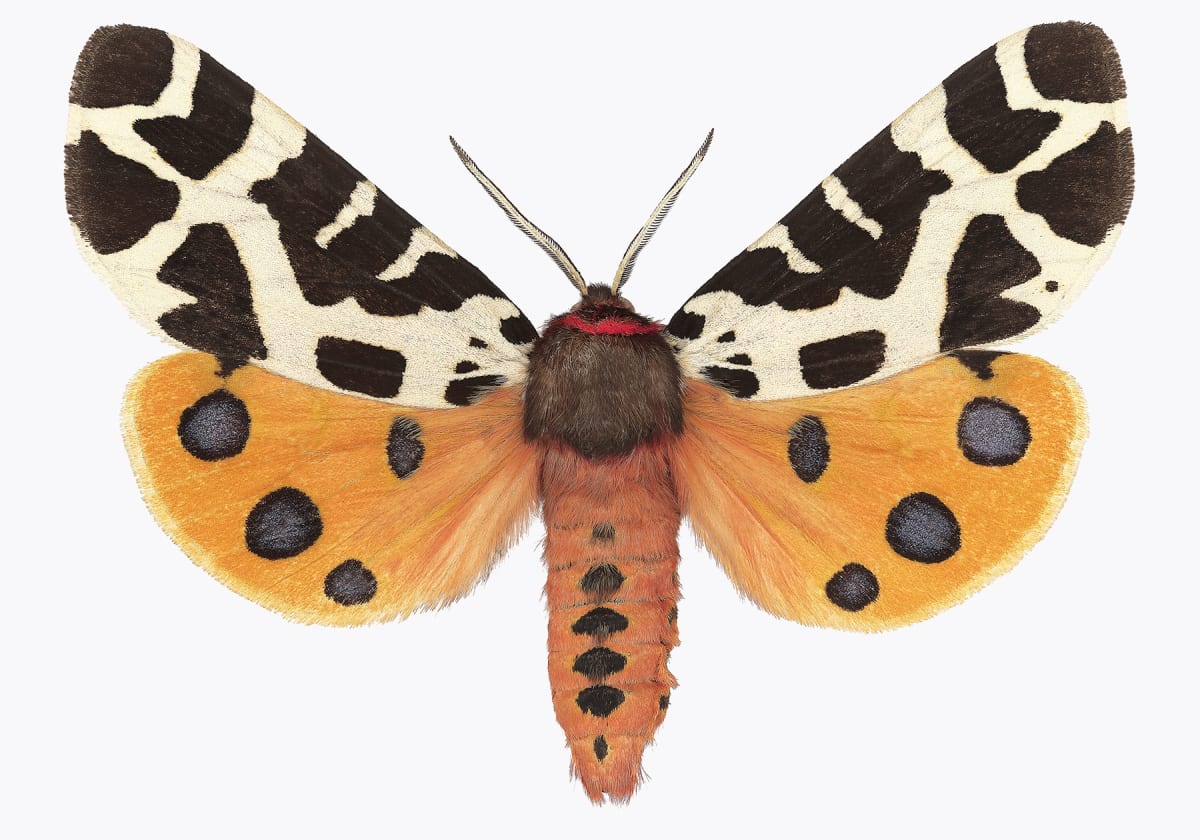A detailed image of a moth on a white background reveals its intricate features. Looking straight down, the moth's wings are spread horizontally. The top pair of wings stretches to the left and right corners, with a white base adorned with random brown inkblot-like spots. The lower pair of wings showcases an orange background interspersed with gray dots and delicate hairs. Notably, each of these wings has three gray dots towards the ends, one with a black circle, and another gray dot at the beginning.
 
The moth's body, centrally located, is large, cylindrical, and somewhat fuzzy. The body's lower part is orange with circular patterns running from top to bottom, accented with black dots across its length. Where the wings meet the body, the central portion is a distinctive brown fuzzy color, transitioning to a darker brown with a hint of red at the head. The moth's light-colored antennas, bordered in black, extend outwards to the left and right from the top of the head, adding to the delicate appearance of this mesmerizing insect.